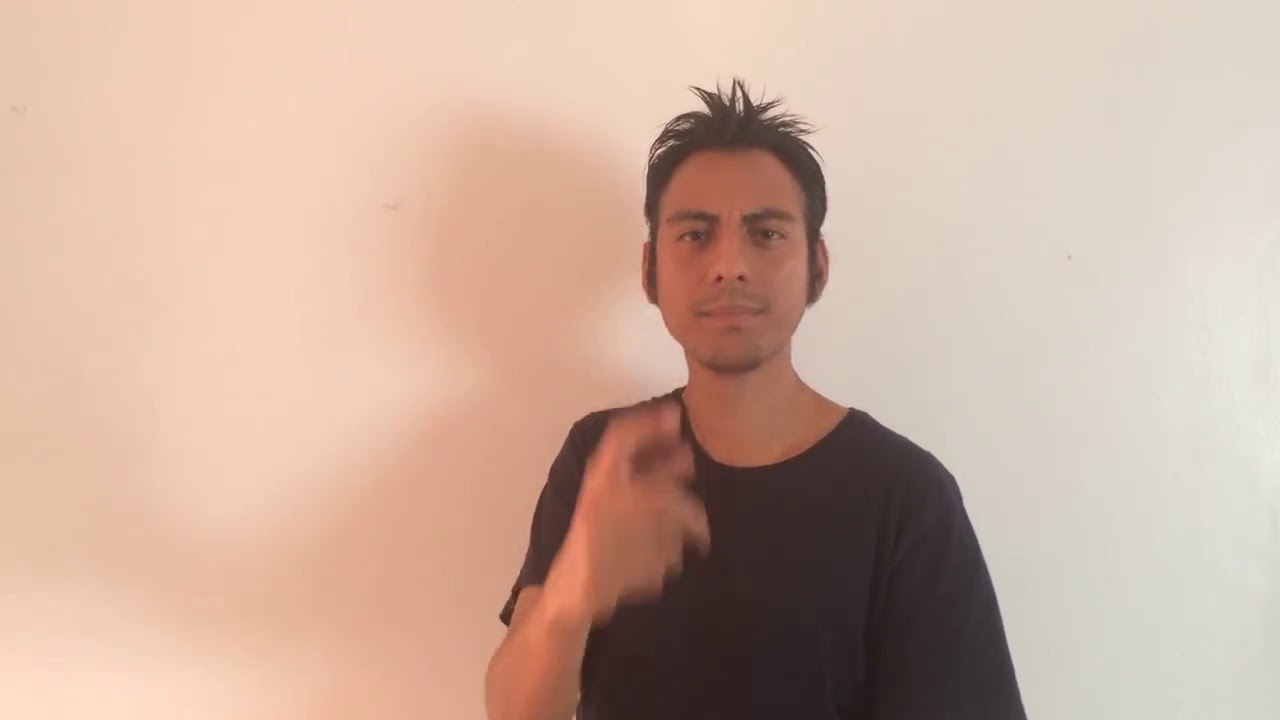In this photograph, a young man, likely in his mid-20s, stands slightly off-center with his body turned towards the camera, giving the impression of being right in the middle of the image. The light behind him casts an orangish-reddish hue due to the lighting conditions, creating a shadow against the whitish, cream-colored wall. He is wearing a black T-shirt and has a tan complexion with short, somewhat spiked black hair and sideburns that extend just past his ears. His facial hair is sparse, featuring a thin goatee and some stubble on his chin and above his lip. The man has his left hand raised and slightly blurred in motion, as though gesturing or pointing with his index finger slightly apart from the rest. He looks straight at the camera, and the setting appears to be indoors, possibly a home or another building. The lighting and shadows are particularly noticeable, adding an interesting depth to the otherwise simple background.